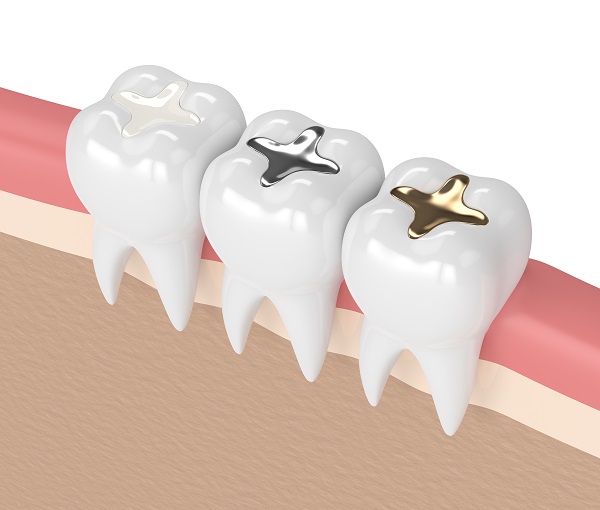The image depicts a detailed diagram of three shiny teeth, each featuring distinct types of fillings. The teeth are positioned on a pink gum surface. Below the gums is a sand-colored layer, and in front of the gums, there is a brown surface. The tooth on the left is topped with a white cross-shaped filling, the middle tooth has a metallic silver cross filling, and the tooth on the right boasts a gold cross filling. The entire ensemble rests against a white background, suggesting a clean and clinical setting, potentially a rendering for dental illustration purposes.